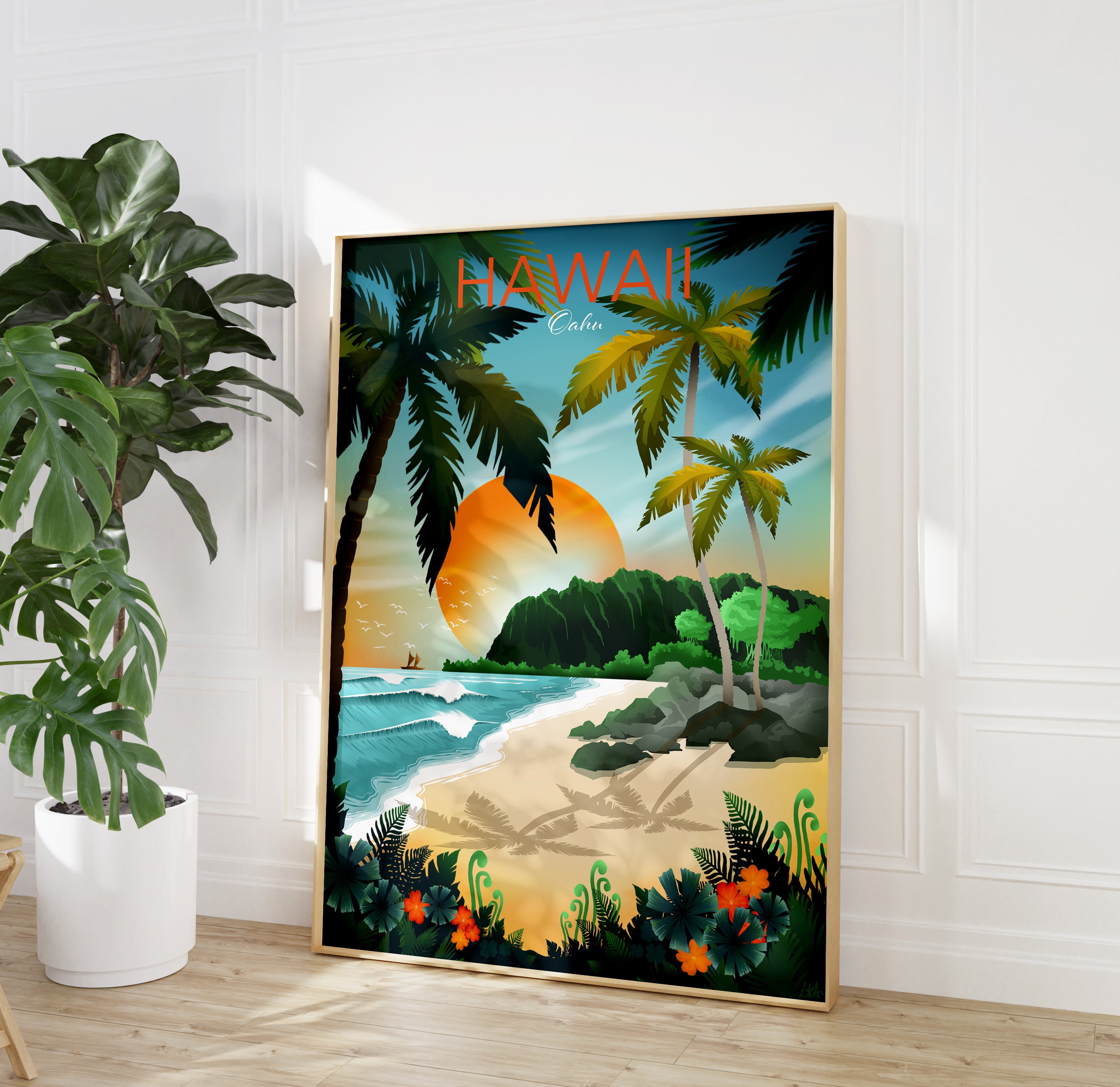The image showcases an elegantly decorated home interior with pristine white walls featuring decorative squares and rectangles, and light oak wood flooring. Dominating the center is a large gold-framed illustration of a scenic Hawaii beach, vividly presenting palm trees, mountains, a radiant sunset, waves crashing onto the shore, and colorful tropical flowers, with the words "Hawaii, Oahu" inscribed at the top. This vibrant artwork leans against the wall, adding a touch of island charm to the room. To the left, a substantial plant with lush green leaves sits in a white pot, while a smaller monstera with fenestrated leaves is partially visible, placed on a wooden plant stand. The ambiance is completed by the subtle presence of a brown table corner in the left portion of the image.